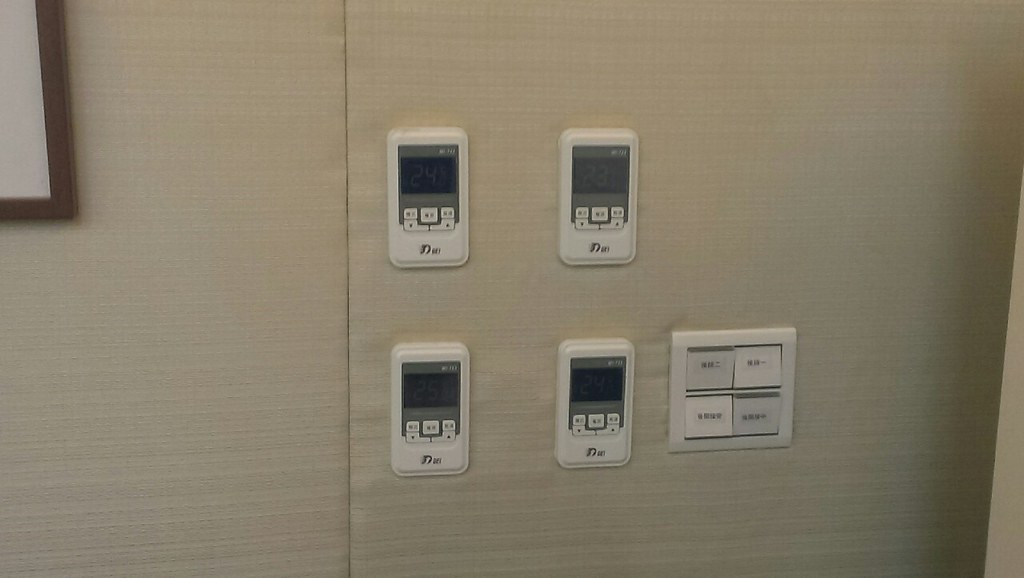The photograph showcases an interior wall of a dwelling, featuring four centrally located devices that appear to be thermostats. Each device resembles a small phone, with the upper third occupied by an analog-like screen displaying information. Beneath the screen, the middle section features several buttons, while the lower portion bears the manufacturer's logo. To the right of these devices are several switches. The textual details on all devices are in either Chinese or Japanese, suggesting the setting may be in an East Asian country. The lighting is diffuse and originates from multiple sources, creating an even illumination across the scene with no visible shadows. On the left edge, a small portion of a framed image is just barely visible, adding a touch of decor to the otherwise plain and utilitarian wall. The image is devoid of people and other textual elements, presenting a clean and straightforward composition.